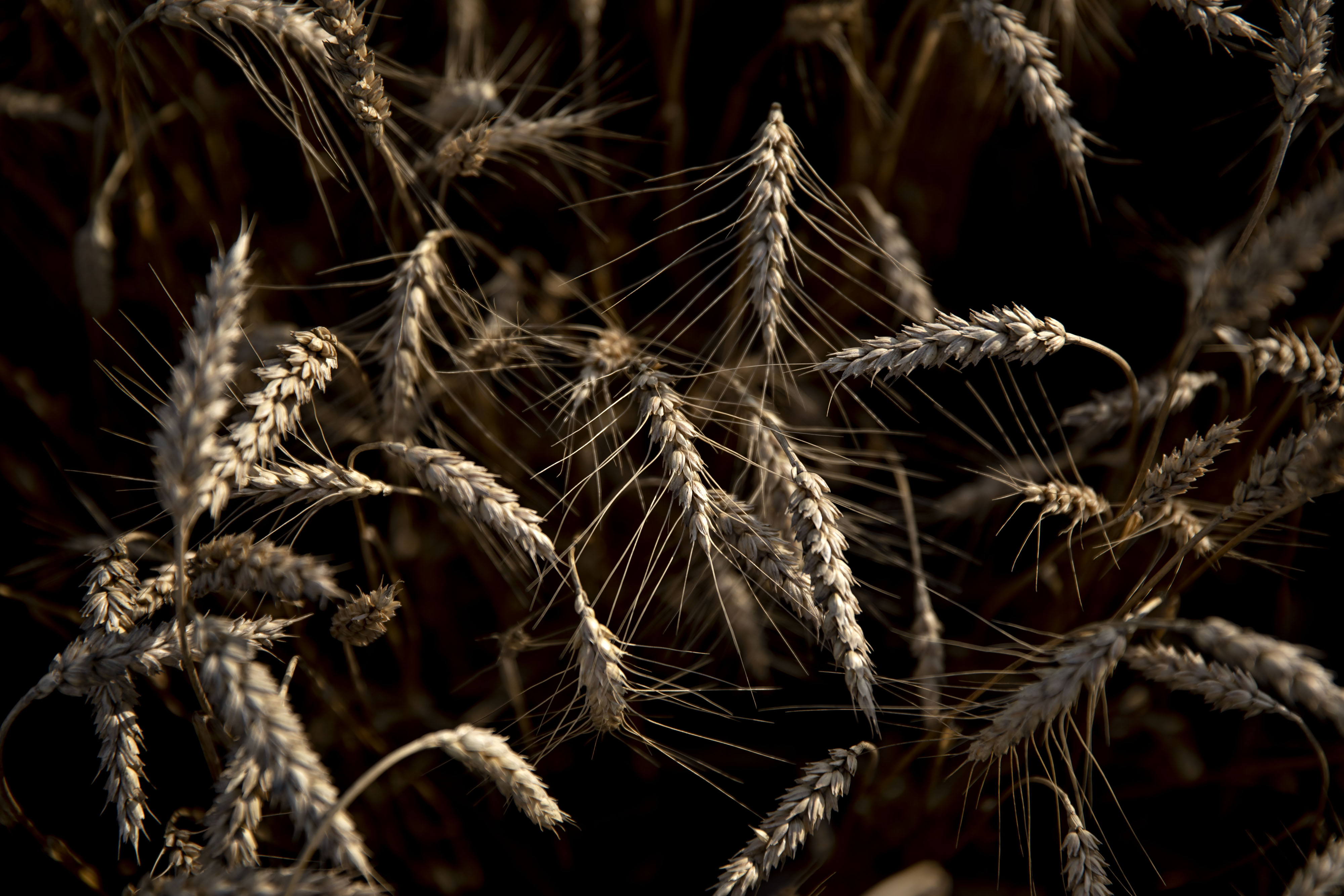The image is a close-up, horizontally-oriented color photograph of the tops of a wheat field, though its appearance suggests it might be computer-generated. The predominant shades are various hues of light brown and beige, contributing to a monotone theme. The foreground displays dried-out, light tan wheat heads with long, thin hairs resembling cat whiskers or bug legs emerging from their bases. These wheat heads are slightly bent and point in various directions, with many appearing to be ripe for harvest. The background, in contrast, is dark and blurred, enhancing the focused, brightly lit wheat chaffs in the foreground, and creating a sense of depth and texture. The overall impression is a field ready for harvest, highlighted by intricate detailing on the primary wheat elements.